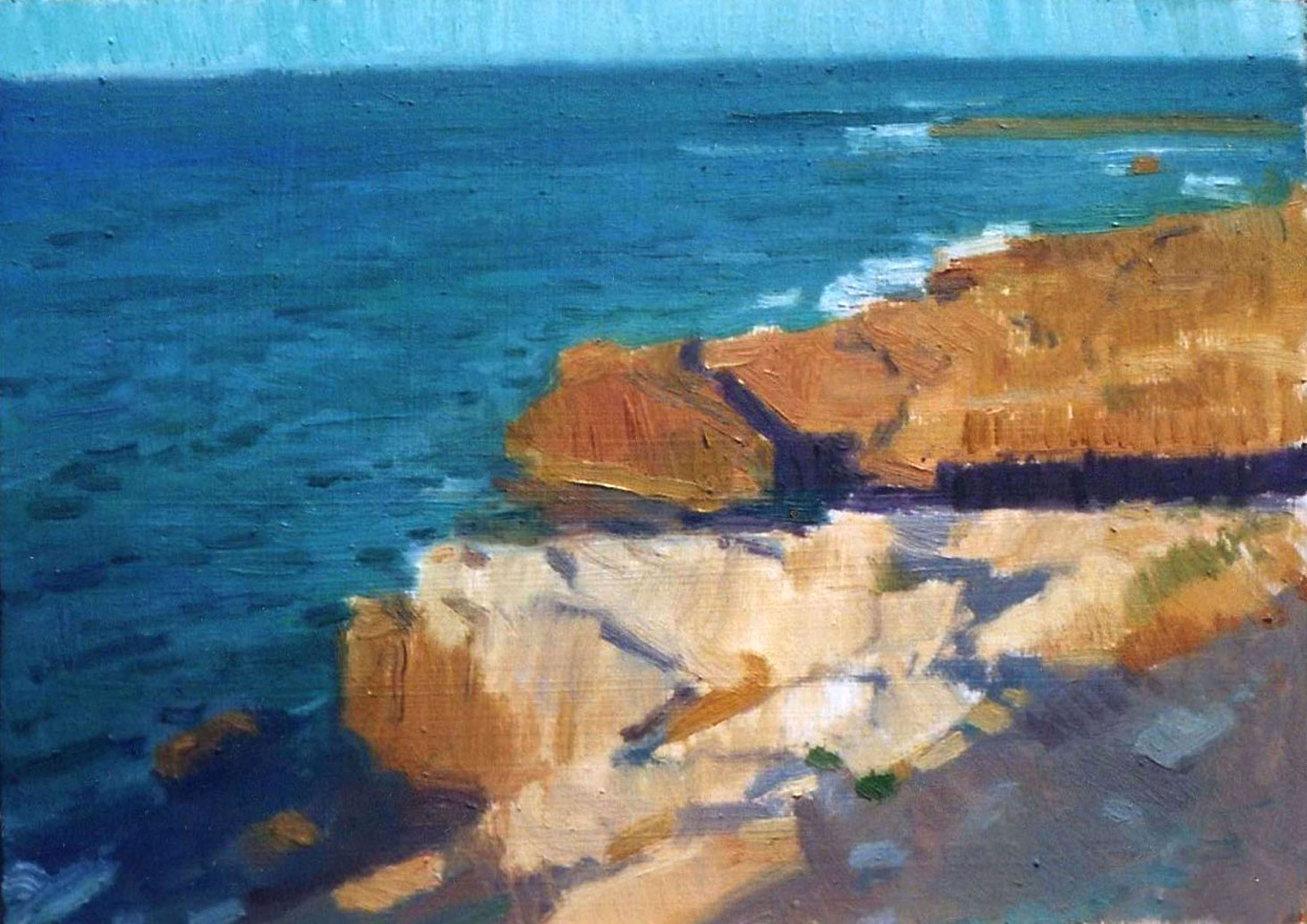The painting depicts a rugged, rocky beach scene, viewed from atop jagged cliffs. The ocean, colored in deep dark blues and teals, stretches across the left side of the image, with small whitecaps indicating where waves meet the shore. High up in the background, the sky is a pale blue, suggesting daytime. The cliffs, primarily brown with sections of white-topped jagged rocks, dominate the majority of the painting. These cliffs appear sharp at their bases, becoming somewhat rounded towards the top, with streaks of blue water interspersed throughout. A small speck of green vegetation grows at the edge of these rocks in the bottom left corner. In the upper right corner is a small brown island or sandbar, surrounded by the continued stretch of ocean. The overall setting feels arid and difficult to traverse, with no trees, flowers, or people present, enhancing the sense of isolation and stark beauty in this natural seascape.